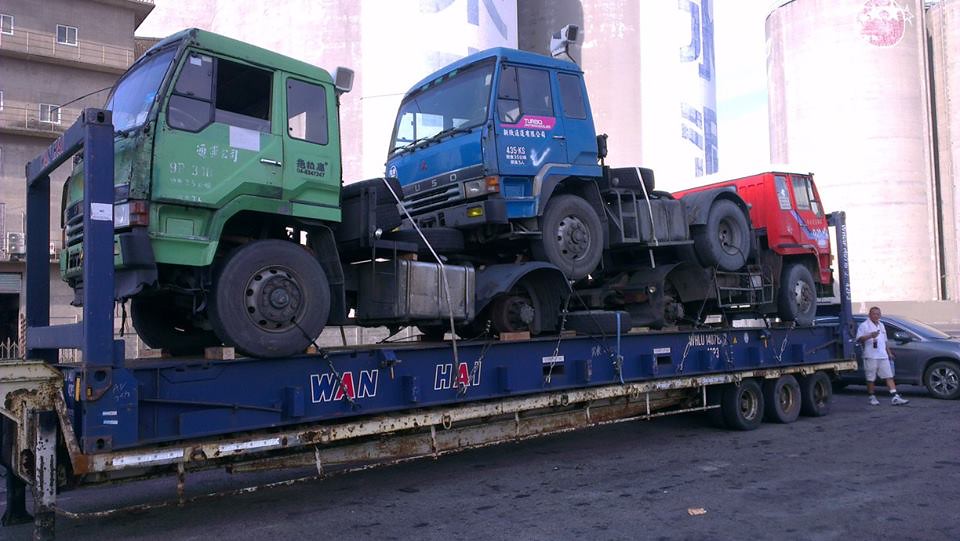In this outdoor daytime scene set in what seems to be an industrial park, a large blue flatbed truck dominates the foreground on a cement road. The truck is marked with the lettering “WANHAI” and has a rusted bottom section and three wheels on the back. It carries three semi-trucks without trailers: a green one positioned on the upper left, a blue one situated further back, and a red one at the rear. A man in a white short-sleeved shirt, tan shorts, and white tennis shoes stands to the right of the truck, holding something in his hand. In the background, tall silo-type buildings and some multi-story structures with faded, blurred colors of white, blue, and red are visible. A car can also be seen at the far end of the road. The scene captures a moment in a city-like, industrial area with a focus on heavy machinery transport.